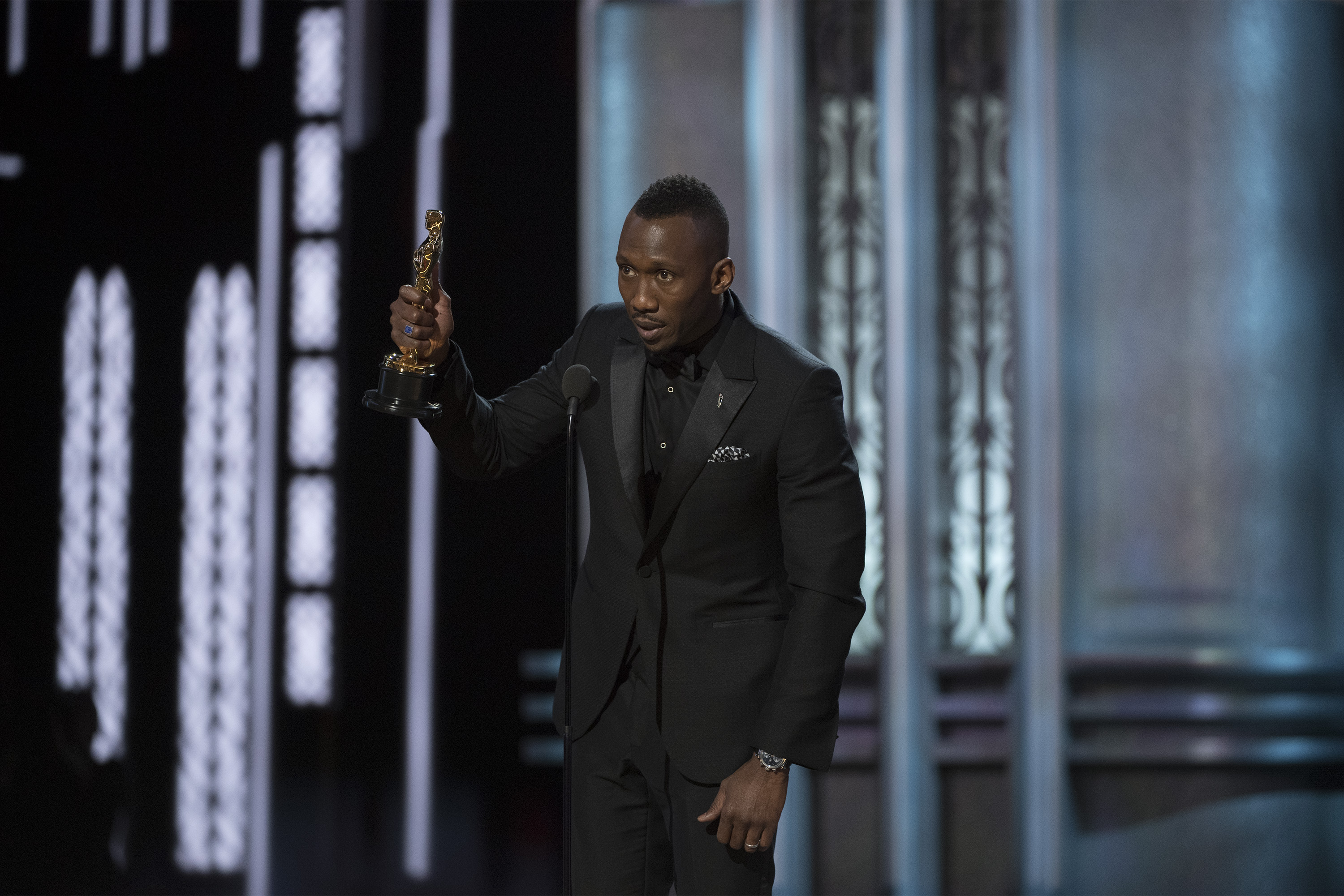The image depicts a black man who has just won an award, likely at the Oscars. He stands alone on stage, addressing the audience with his mouth partially open as if speaking into a standing black microphone. He is elegantly dressed in a black tuxedo, complete with a black shirt, black bow tie, and a white polka-dotted handkerchief in his breast pocket. He wears a watch and a wedding ring on his left hand, which rests at his side, while his right hand is raised, proudly holding a trophy resembling a human figure perched on a black base. He has short black hair and a bit of a mustache. The backdrop of the stage features a striking combination of silver columns and window-like structures, interspersed with dark sections, creating a dramatic visual effect. The floor beneath him is dark, accentuating the luminous elements behind. The image is wider than it is tall, capturing the grandeur and poise of the moment.